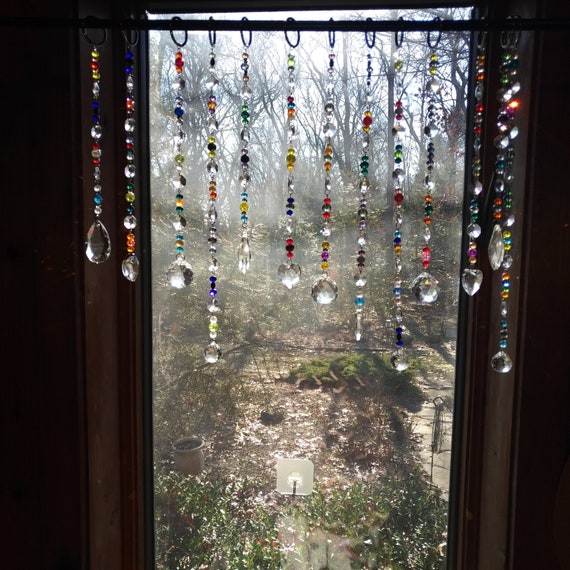This photo captures a view from inside a building, looking out through a large window into a garden area. The window, outlined by its frame, showcases an array of decorative light catchers hanging from a curtain rod across its top. These strands of colorful glass beads, about a dozen in number, extend partway down the window in slightly varied lengths, each culminating in a larger clear bead. The sunlight pours through the glass, catching and shimmering on the beads, casting beautiful light patterns inside. Outside the window, the garden appears somewhat untended with patches of dry dirt and sporadic greenery, a couple of small plants and paving stones scattered about. In the background, tall barren trees devoid of leaves stand starkly against the sky, framing the wild, rustic scene.